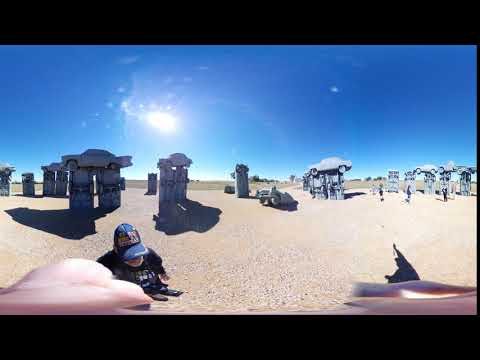The image depicts the iconic Carhenge, an automotive parody of Stonehenge, set in a desolate, cracked dirt landscape resembling a desert. In the background, multiple stone-like or metallic vehicular structures are perched atop tall stone pillars, with seven or eight of these pillars supporting car-shaped constructs. A few pillars remain unadorned. In the lower left quadrant of the photo, the upper half of a man wearing a blue baseball cap and a black t-shirt is visible. The horizon divides this extraordinary scene from a bright blue, cloudless sky above. There is a noticeable sun flare in the upper left quadrant of the image, possibly reflecting off a dirty camera lens. Additionally, distorted flesh-colored shapes, likely fingers, obscure the bottom corners of the photo, contributing to the overall surreal and artistic ambiance of the display.